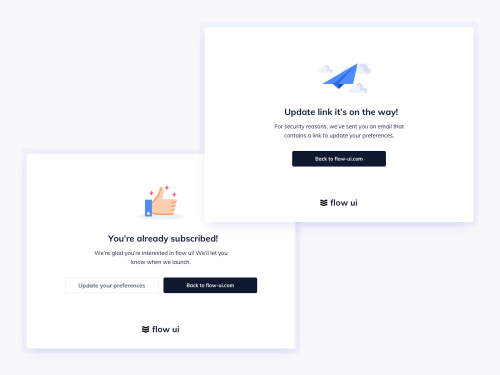This image is a compilation of two separate photographs centered around user interaction with the Flow UI platform. 

The first photo prominently features a thumbs-up emoji paired with three red diamond emojis, accompanied by the text: "You're already subscribed. We're glad you're interested in Flow UI. We'll let you know when we launch." Below this message, there are two buttons: one with a white background labeled "Update your preferences," and another with a black background labeled "Back to flowai.com." At the bottom of the image, the words "Flow UI" are displayed alongside a black icon resembling a small square. The overall background is white with black text, punctuated by colorful emojis.

The second photo features a blue paper plane set against gray clouds and conveys the message: "Update link is on the way. For security reasons, we've sent you an email that contains a link to update your preferences." This image also includes a button with a black background labeled "Back to flowui.com." Similar to the first photo, the name "Flow UI" and its corresponding square-shaped black icon are positioned at the bottom. The background remains white with black text, enhanced with various colorful emojis. The entire composition is set against a gray background, providing a cohesive and visually engaging presentation.